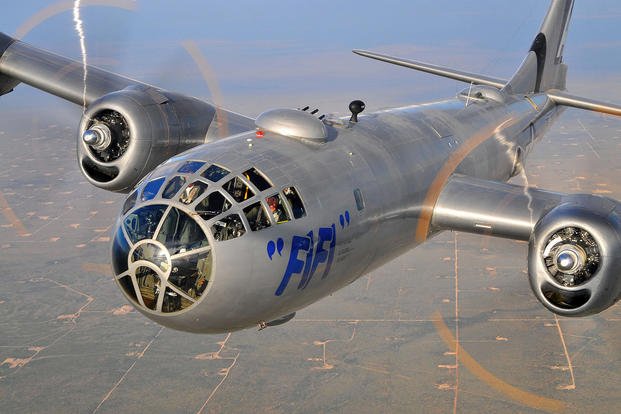This photograph features a vintage airplane in mid-flight, prominently filling the frame against a backdrop of distant fields and roads below. The aircraft is reminiscent of designs from the 1950s or 1960s, characterized by its rounded, silver-colored body crafted from stainless steel. The nose of the plane is distinctly oval, showcasing a large glass cockpit segmented into five sections with an additional central circular window, allowing a clear view inside. The propellers, attached to engines on either wing, are visibly spinning at high speed, leaving behind an orange hue. The aircraft bears blue painted characters "V.F.E." on its side, although another caption mentions it as "F.I.F.I." suggesting it might be military-style. Atop the plane, a notable metallic feature with three protruding pipes and a camera-like structure can be seen. The photo captures the aircraft against a wide, high-altitude expanse, underlining its graceful, iconic mid-century design.